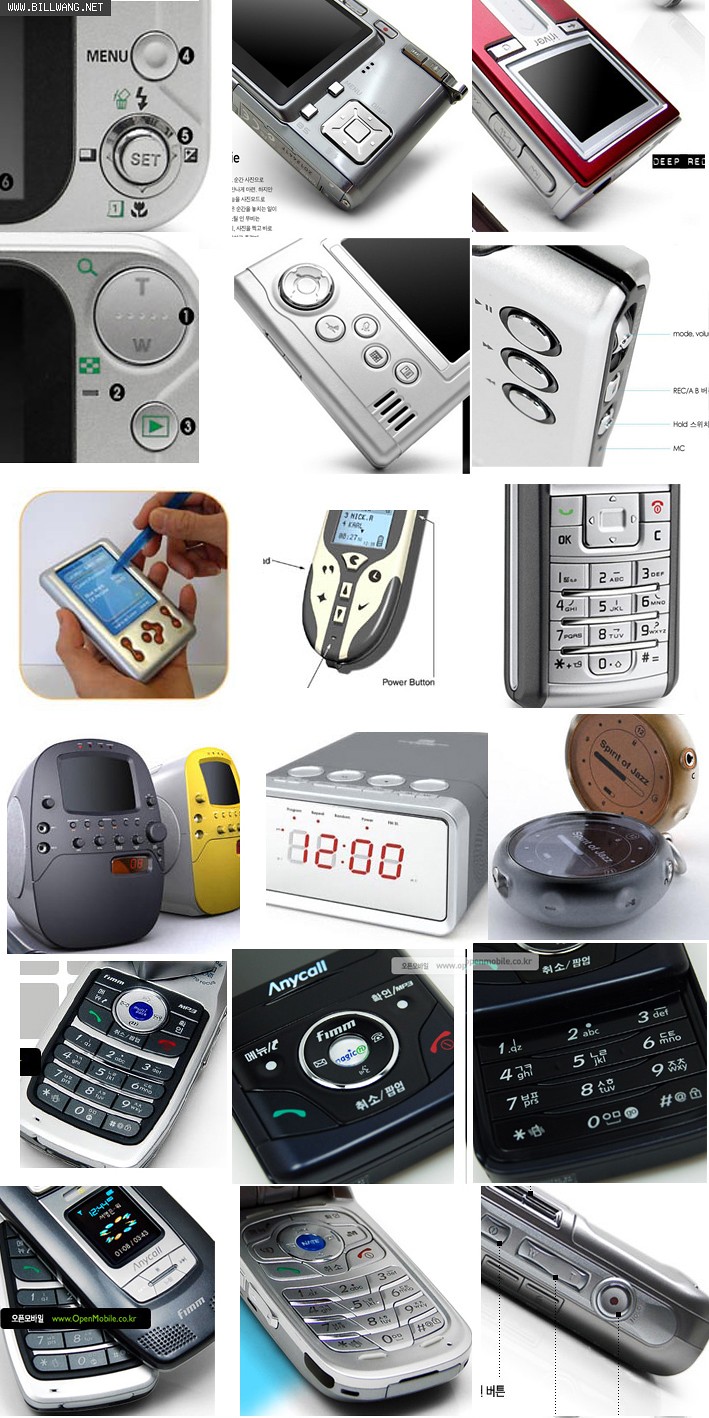The image is a detailed, 18-photo montage showcasing close-ups of various electronic devices. Each square image captures elements like buttons, switches, and screens. The items include MP3 players, digital cameras, clocks, remote controls, small television sets, cordless telephones, old cell phones, radios, and alarm clocks. Many have buttons with Chinese characters. The montage also features flip phones, some silver and some black with "Anycall" branding, and a cell phone with a light blue stylus. The central image is an alarm clock. The emphasis is on the intricate details of these everyday electronics, presenting a colorful and nostalgic collection of technological interfaces.